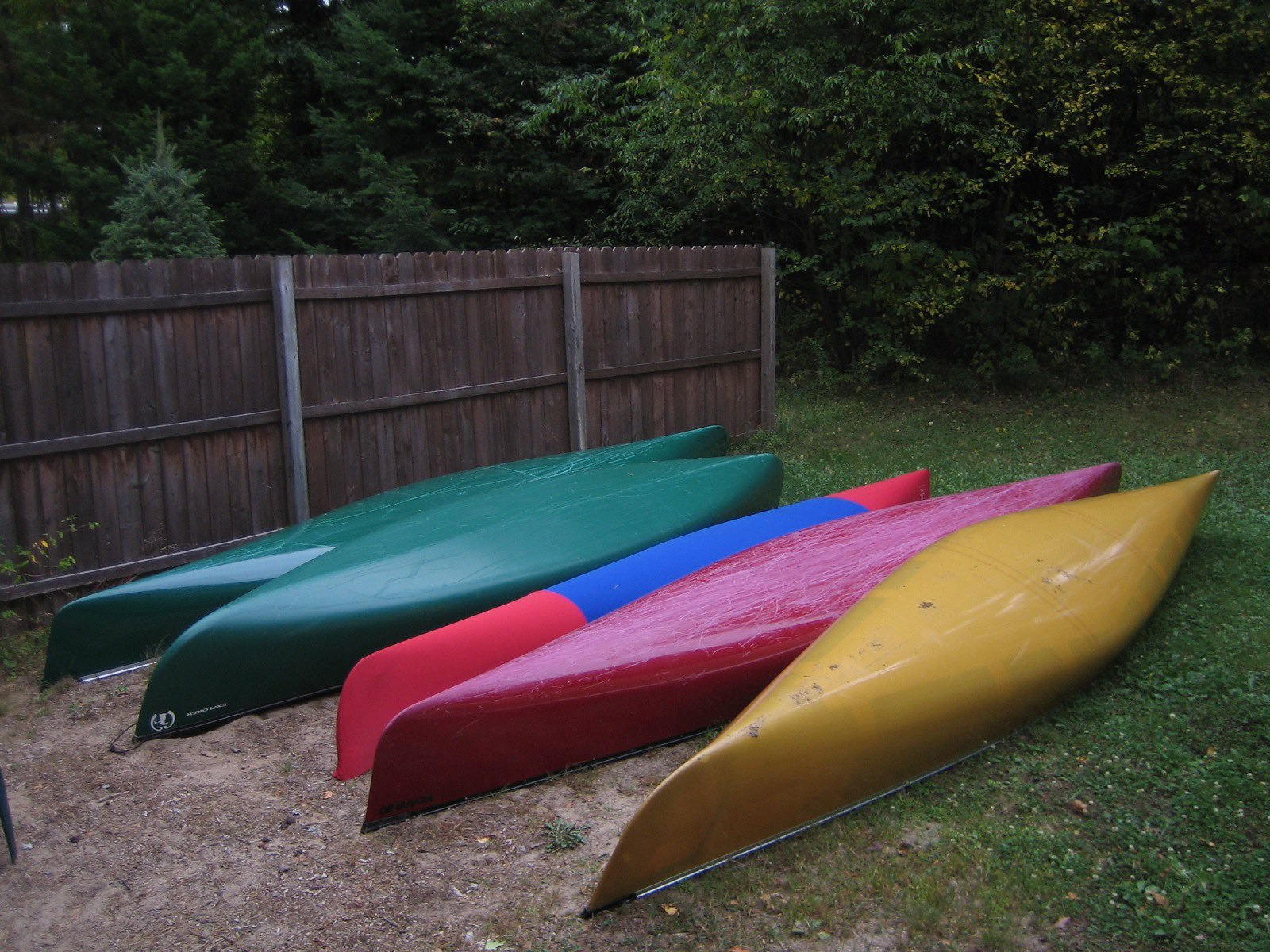In this outdoor photograph, five canoes are positioned upside down and leaning against each other next to a weathered wooden fence comprised of three sections. Nestled in a mostly grassy clearing, the canoes display a variety of colors: two with green bottoms, one in amber, one with a magenta-reddish hue marked with scratches, and another with a striking blue middle flanked by orange (or light red) ends. Behind the fence, a pine or spruce tree stands prominently, accompanied by other trees that extend into the distance. The area transitions from dirt in the front left to grass and moss towards the back and right, with the overall scene evoking the calm, rustic charm of a park or possibly a spacious backyard.